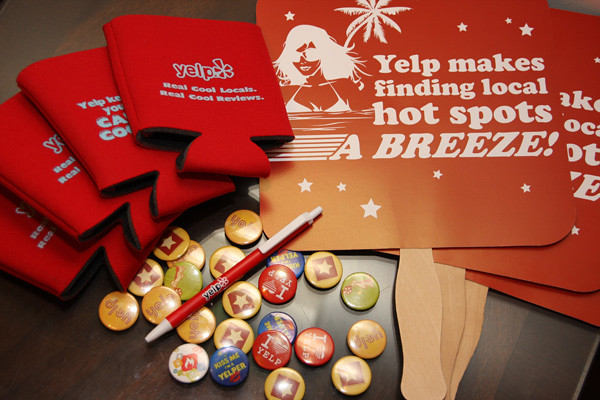The photograph showcases a table laden with promotional items, likely intended as conference swag. On the top left are four red drink koozies, neatly fanned out, each adorned with white text saying "Yelp. Real cool locals, real cool reviews." To the right, there are three red paddles resembling signs on plain wooden sticks. Each paddle features a design of a woman in sunglasses and a palm tree, with additional white stars and the text "Yelp makes finding local hotspots a breeze."

At the bottom of the image, a mix of colorful pins is scattered across the brown table surface. The pins include red ones that say "I ♥ Yelp," blue ones with "Kiss me, I think I'm a Yelper" and a lip print, and yellow ones featuring a star design. Overall, there appear to be approximately 15 to 20 small buttons. Dominating this array of pins is a red and white writing pen, prominently branded with the word "Yelp."